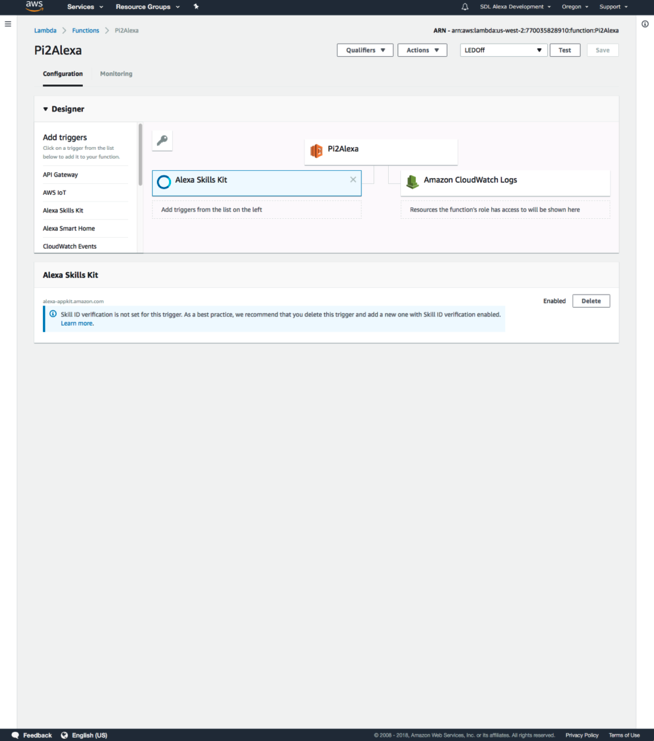The image displays an Amazon Web Services (AWS) interface. In the top left corner, the AWS logo is shown prominently, featuring the iconic orange smile design with "AWS" written in white against a black background. The top portion of the image includes a navigation bar with tabs labeled "Services," "Resource Groups," and an icon for pins. 

On the top right, the interface lists various categories such as "SDL," "Alexa," "Development," and "Support." 

Along the left side, there's a text label "lambda function: pi2alexa," with subcategories for "Configuration" and "Monitoring"; "Configuration" is highlighted. Below this, tabs labeled "Designer," "Add triggers," "API Gateway," "AWSIoT," "Alexa Skill Kit," "Alexa Smart Home," and "CloudWatch Event" are visible.

Adjacent to these tabs, on the right, "Alexa Skill Kit" is noted alongside a blue settings icon. Instructions to "Add triggers from the list on the left" are displayed, followed by "pi2alexa" at the top. To the right of these instructions, "Amazon CloudWatch Logs" is mentioned. 

A flow diagram in the center traces a path from "pi2alexa" at the top to "Alexa Skill Kit" on the left and "Amazon CloudWatch" on the right. At the bottom of the image, there's a notation about Alexa Skill Set, reminding users that "Skill ID verification is not set for this trigger. As a best practice, we recommend that you delete this trigger and add a new one with Skill ID verification enabled." A "Learn More" link, highlighted in blue, provides additional information. Two white buttons labeled "Enable" and "Delete" are located on the right side of the image.